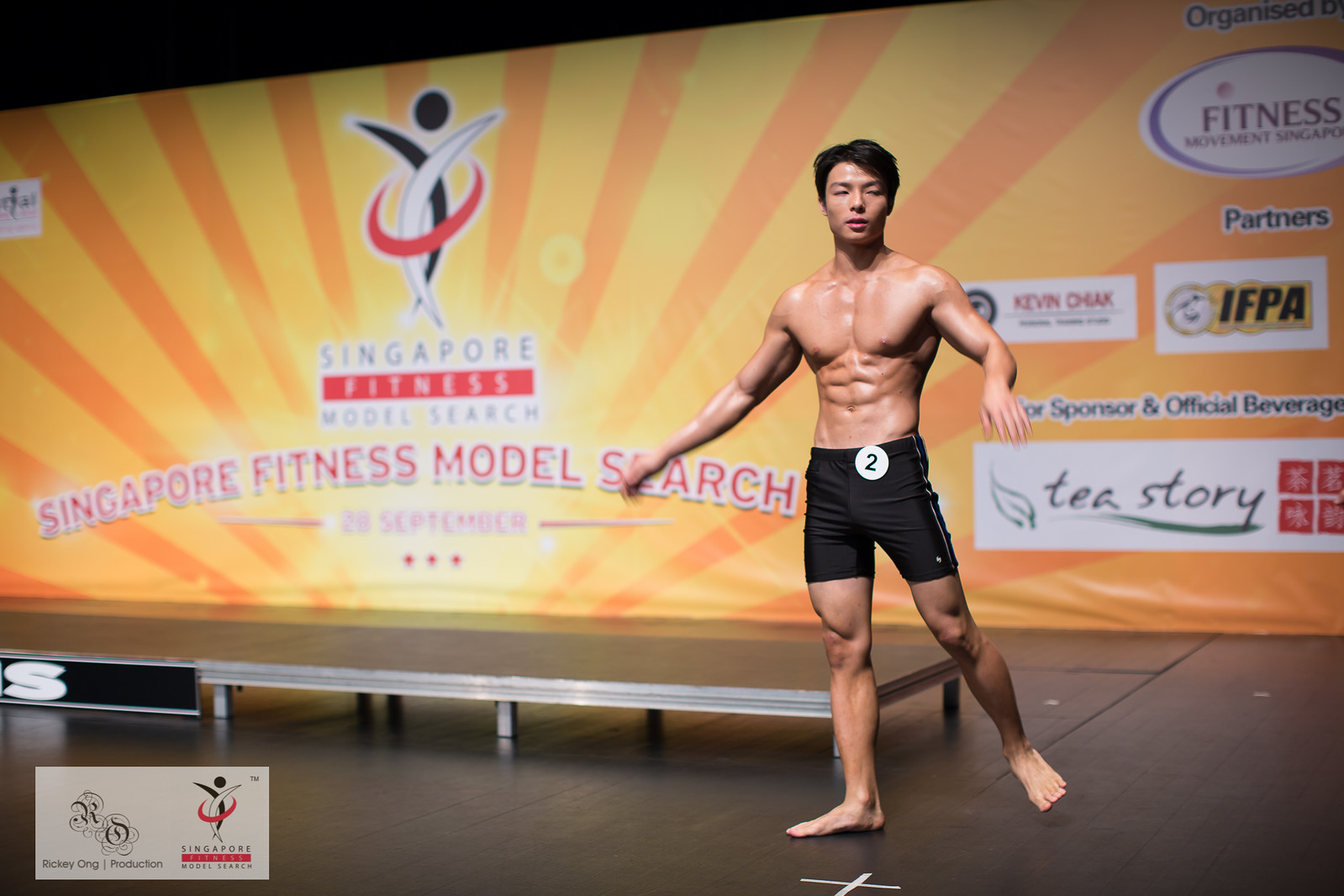This photograph showcases a very fit and muscular young Asian man posing barefoot in tight black shorts with a white number two on their waistband, indicating he is the second competitor. He has black hair and is in a dynamic stance, with his arms appearing to swing as they exhibit motion blur. The setting is a wooden floor marked with a taped "X" on which he stands, suggesting a designated spot possibly for runway or stage presentation purposes. In the background, there's a vibrant yellow and orange sunburst banner featuring the event's name, "Singapore Fitness Model Search," displayed prominently in red and white text. The banner also shows the event date, 28th September, although it is slightly blurry. The right side of the banner is adorned with numerous sponsor logos, including Tea Story, IFPA, Kevin, Chak, and Fitness, alongside a small emblem resembling a person designed with swirl lines at the bottom left corner. The surroundings and details strongly indicate that this scene is part of a fitness model search competition in Singapore.